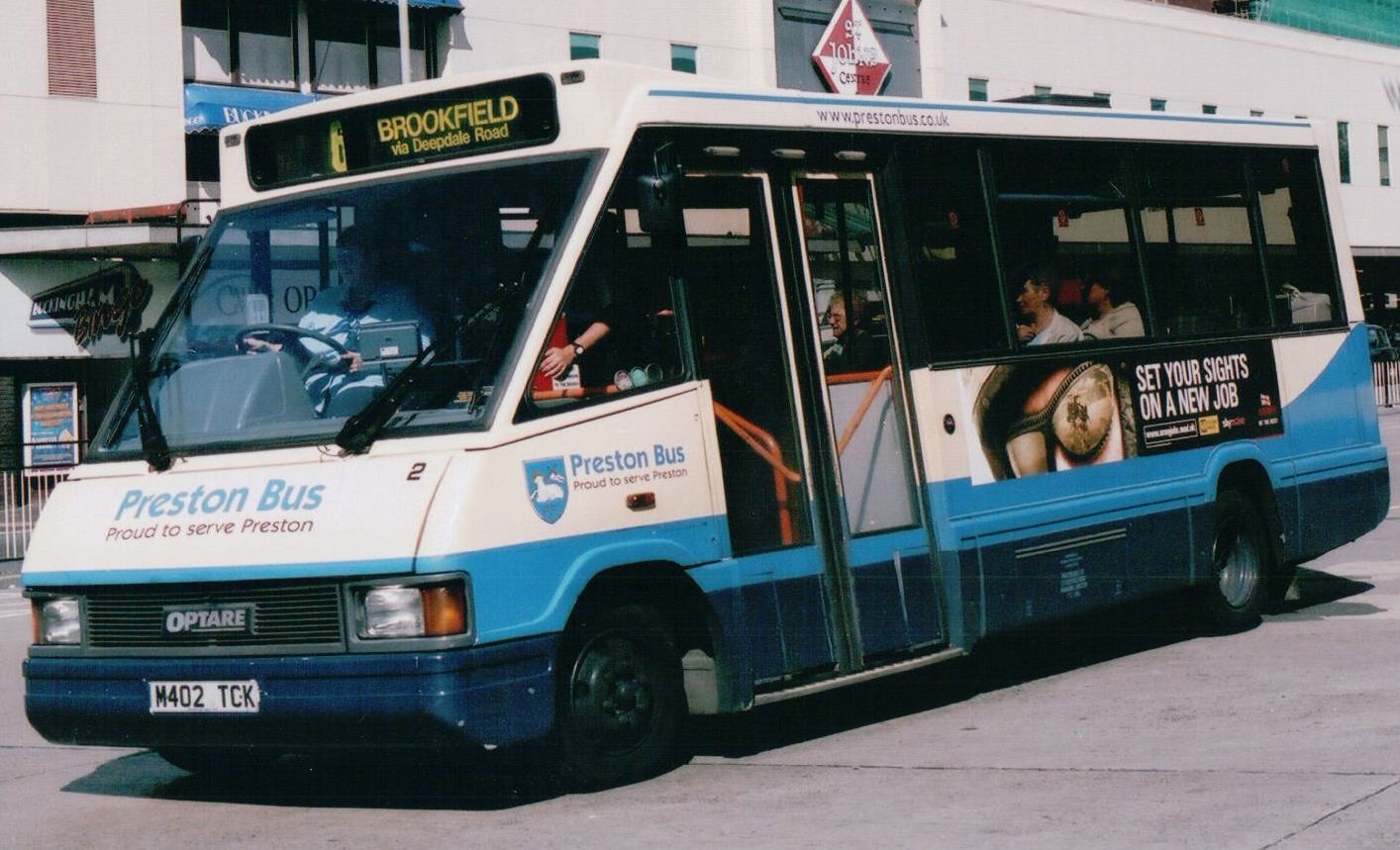The photograph is an outdoor scene taken during the daytime, featuring a rectangular, single-decker shuttle bus with an older design. The bus has a pointed, slanted windshield at the front, giving it a triangular look, and the rest of the bus is rectangular. The front and right-hand side of the bus are visible. A black oval sign with yellow text at the top front of the bus reads "6, Brookfield via Deepdale Road" and "Preston Bus, proud to serve" is printed in blue on the hood and in red below. The license plate is "M402 TCK." The bus exterior is primarily white, with a light blue band just above the wheels and a darker blue section at the bottom. 

The bus is occupied, but not full. A driver is visible on the left, wearing a white shirt, and a person stands beside the bus, presumably waiting for the double doors to open. An advertisement on the right side of the bus reads, "Set your sights on a new job," accompanied by an image of a man with glasses. Above the windows on the side of the bus is the URL "www.prestonbus.co.uk."

The background shows a row of two-story buildings with multiple windows and a road made of large gray cement blocks. In the center of the background, a red and white diamond sign, possibly saying "Jobeva Castle," is visible.